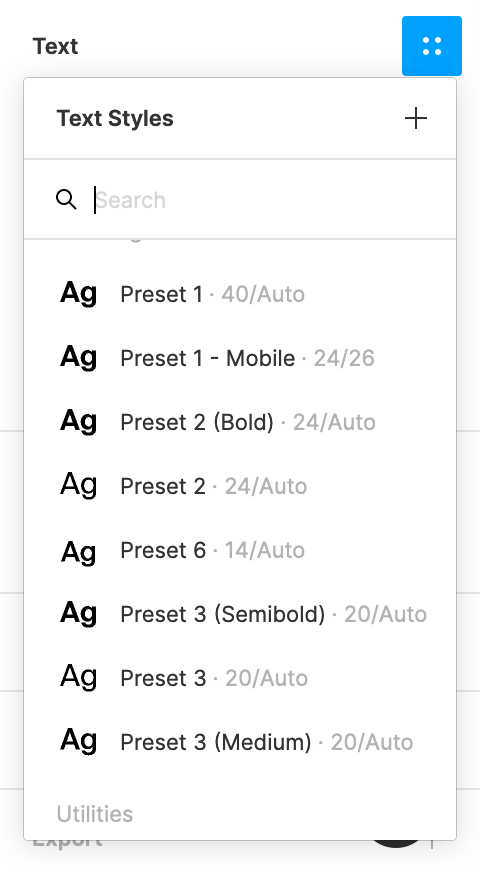This image is a screenshot of a "Text Settings" dialog box. In the top left corner, the heading "Text Styles" is prominently displayed. Directly below this heading, there is a search bar for filtering text styles. To the right of the search bar, there is a plus symbol icon, which allows users to add new text styles. The central area of the dialog box features a large dropdown menu containing various text style presets, each represented with the abbreviation "AG."

Below is a detailed list of available text styles within the dropdown menu:
- Preset 1
- Preset Mobile 1
- Preset 2 Bold
- Preset 2
- Preset 6
- Preset 3 Semi Bold
- Preset 3 20/Auto
- Preset 3 Medium

In the bottom right corner of the dialog box, the word "Utilities" is displayed, likely signaling additional functions or tools related to text settings. The entire interface has a clean, minimalist design with a white background and black letters, ensuring clear readability of the text.